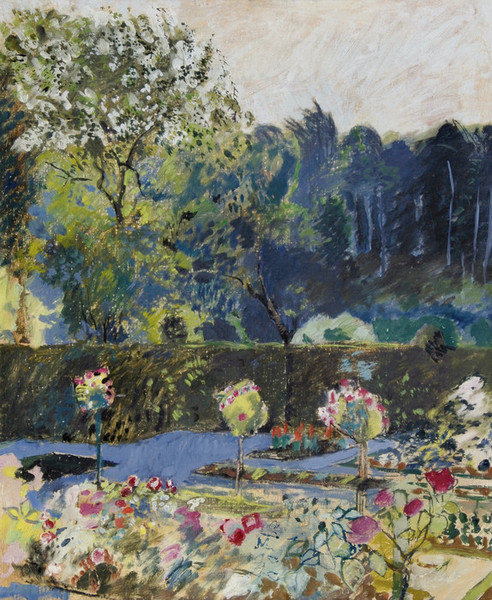This painting, which evokes a style reminiscent of Monet, portrays a serene outdoor garden scene rendered in watercolors. The foreground features an array of loosely sketched, vibrant flowers in pink, white, yellow, and various other colors. These flowers are interspersed among mini trees with long stems and green, cotton candy-like foliage. The arrangement resembles long, multicolored rectangular tables topped with these florid bushes. Also visible close up are clusters of orange flowers with green petals. 

In the middle of the composition, a continuous hedge wall stretches horizontally from left to right, made up of rich green hues. This boundary leads the eye further back to an area filled with more trees, which are suggested through dark, bluish shapes and gentle outlines. The background comprises an off-white, beige-toned sky, contributing to the overall peaceful and happy atmosphere. Notably, the painting also features water elements, suggested by blue watercolor areas around the flower arrangements, enhancing the tranquil feeling of the scene. No creatures or signatures are visible, solely the lush natural elements.